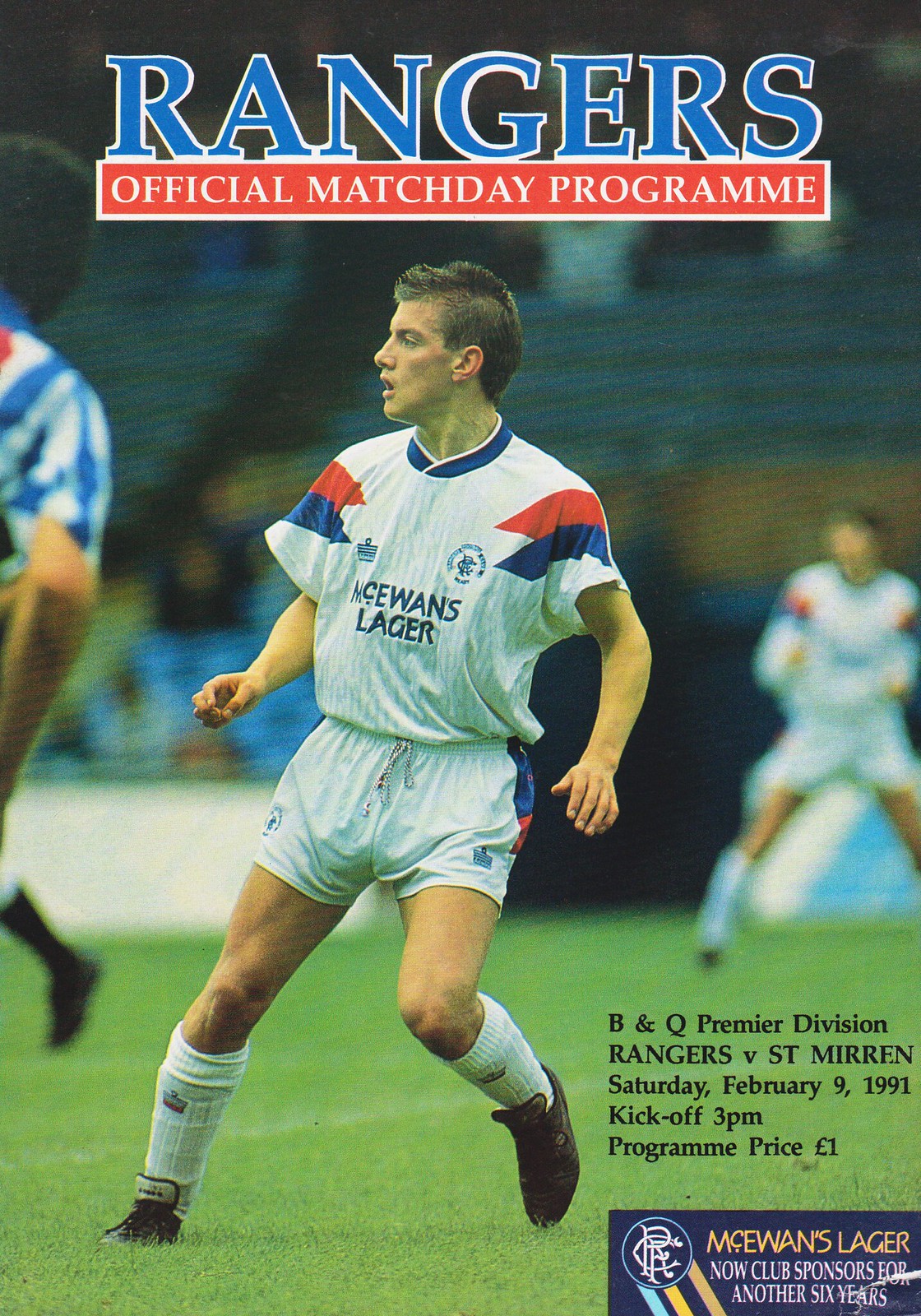This is a detailed photograph of the front cover of a sports program poster, specifically for a soccer match. The main focus is a central image of a Caucasian soccer player mid-action, appearing surprised, and wearing a white uniform with distinctive red and blue stripes along the sides of his shorts and shoulders. The player is donned in white socks and black shoes, and the front of his shirt features the logo for McEwan's Lager. Blurred in the background are other players and likely spectators seated on bleachers, with the green grass field visible underfoot. 

The top of the poster prominently displays the title "Rangers Official Match Day Program" in blue capital letters. Below this title, in a red box, it reads "Official Match Day Program." The bottom section provides detailed event information in black text: "B&Q Premier Division, Rangers vs. St. Mirren, Saturday, February 9, 1991, Kick-off, 3 p.m., Program Price, 1 Euro." Additionally, a small navy blue rectangle at the bottom mentions, "McEwan's Lager now club sponsors for another six years."